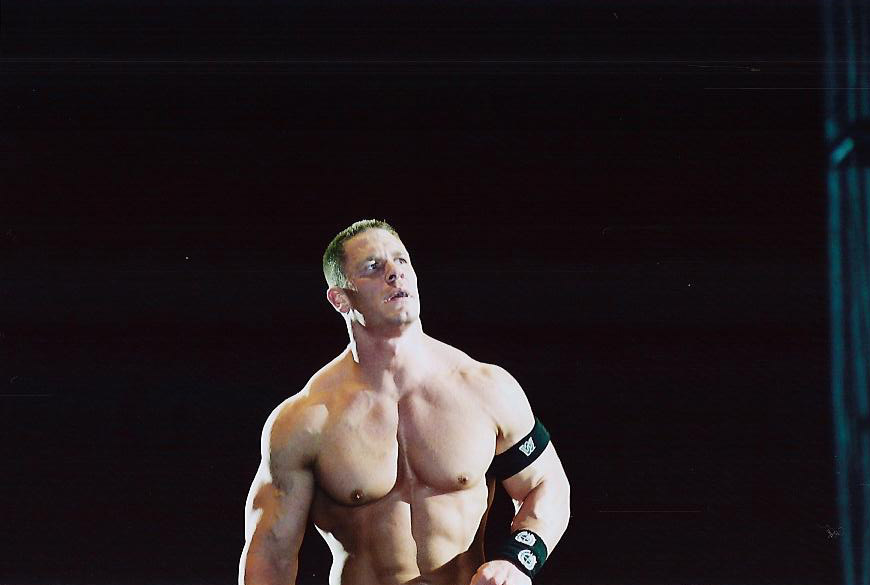This photograph features a shirtless, muscular Caucasian man with short blonde-brownish hair. His impressive physique is highlighted by well-defined chest and arm muscles, suggesting he might be a bodybuilder. The man wears a black sweatband with a WWE logo around his bicep and two black wristbands, each with a white logo on them, around his wrists. He is standing against a completely black background, with his eyes looking upward and to the left. His nipples are a darker brown, and there appears to be some kind of black metal bar on the right side of the image.